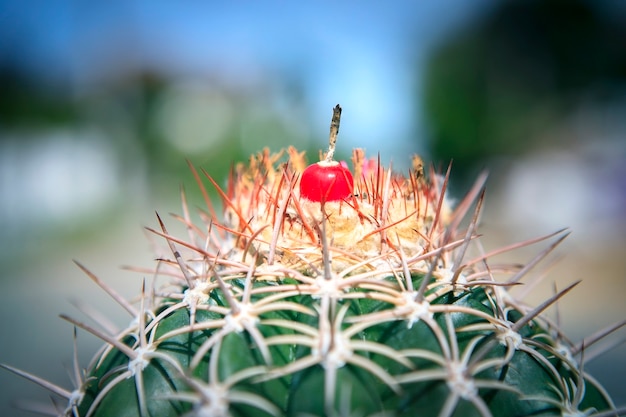This is a close-up photograph of a green cactus taken outdoors. The bottom part of the image showcases the top of the cactus in an arch shape, revealing its succulent, green flesh. The cactus is densely covered with tan or off-white spikes that resemble tiny spidery formations or floral shapes, each originating from small, circular, wood-colored bases. These spikes are connected to the plant by what looks like leafy structures, adding to the intricate pattern. At the apex of the cactus, there's a striking array of spikes that transition from tan at the base to red and purple at the tips. Dominating the center is a vivid cherry-red ball, reminiscent of a cherry tomato but actually a part of the cactus, with a dark, protruding stem. The background is artistically blurred, featuring muted greens, whites, and hints of brown, creating a beautiful contrast that emphasizes the intricate details and vibrant colors of the cactus itself.